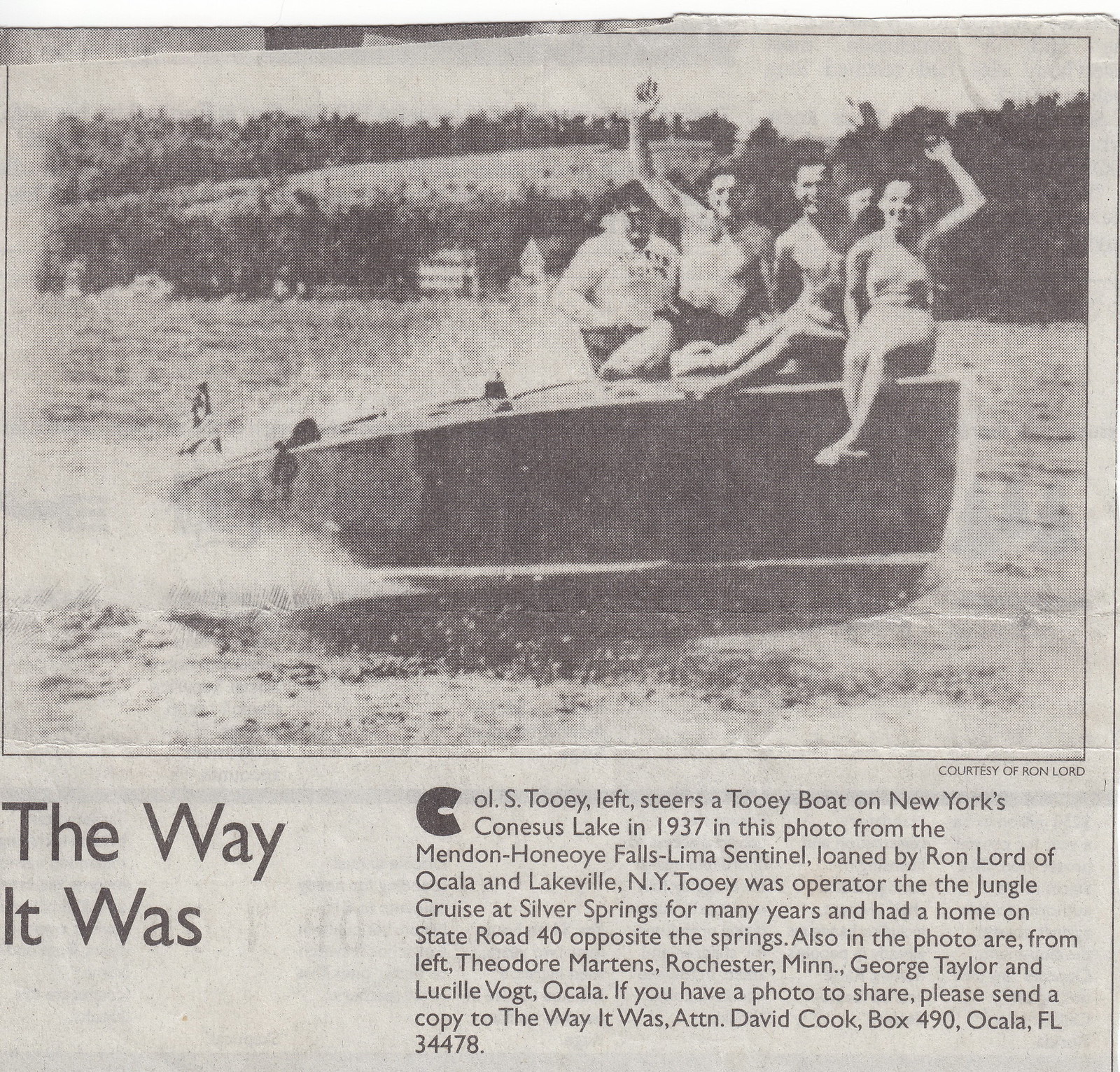This image is an old newspaper clipping titled "The Way It Was," featuring a 1937 black and white photograph from the Mendon-Honeoye Falls Lima Sentinel, loaned by Ron Lord of Ocala and Lakeville, New York. The faded, low-resolution photo shows a scene on New York's Conesus Lake. Colonel S. Tuohy, left, is seen steering a motorboat, with water splashing behind it. Around him, three men and a woman sit in swimsuits and trunks, waving as the boat moves. The background faintly reveals trees and a hillside. Also identified are Theodore Martins of Rochester, Minnesota, George Taylor, and Lucille Vogt of Ocala. Tuohy, known for operating the Jungle Cruise at Silver Springs, lived on State Road 40 opposite the spring.